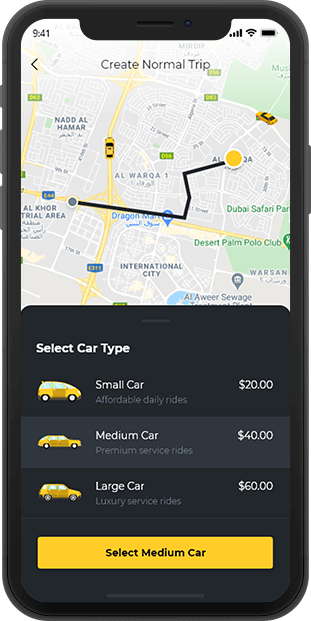The image displays a user’s black cell phone encased in a dark gray or black protective cover. The phone screen reveals the user is in the process of creating a reservation for a ride. At the top left corner of the screen, the time is displayed as 9:41 in black text. To the right, there is an indication of five full bars of network signal and a full battery icon.

The upper half of the screen features a map on a gray background, illustrating the user's current location and intended destination. The roads on the map are delineated in white, with a few green spaces indicating parks or similar areas. A black line marks the route from the starting point to the destination.

The lower half of the screen has a solid black background with white text. At the top, "Select Car Type" is prominently displayed. Below this, a vertical list of three car options is presented, beginning with the "Small Car" option on a light gray background, signifying its selection. This option includes an image of a compact gold car, a description in tiny gray text reading "Affordable daily rides," and a price of $20 in white text.

The second option, "Medium Car," shows a medium-sized sedan with a description in gray text, "Premium service rides," and a cost of $40 in white text. Finally, the "Large Car" option lists a luxury car, described in gray text as "Luxury service rides," priced at $60.

At the bottom of the screen, a prominent bright yellow button reads "Select Medium Car" in black text, indicating the user’s intention to choose the medium car option.